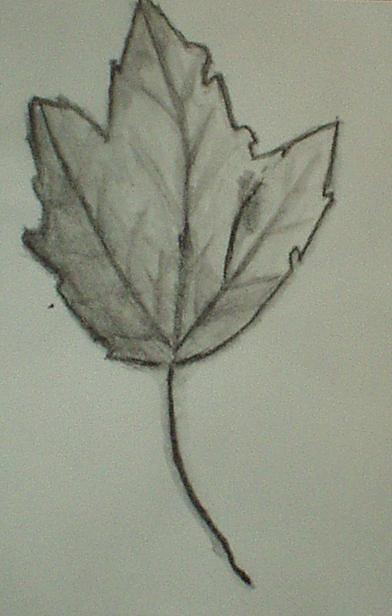This is a black and white sketch of a maple leaf, drawn with pencil on an off-white, almost gray sheet of paper. The leaf, roughly 2 1⁄2 to 3 times taller than it is wide, features a long stem that arcs starting about two-thirds over from the left and extends roughly toward 45% up the page, curving to the right. The maple leaf, slightly jagged and not perfectly symmetrical, has three main points: one at the top and two out to the sides, with an additional spike on the right. The leaf displays distinct veins that branch out towards each point, adding detail and texture. The shading, primarily on the left side, complements the veins and adds depth to the drawing. Some areas appear smudged, possibly intentionally, extending a gray tint beyond the leaf's borders. The drawing exudes a simplistic, natural feel, enhanced by the subtle gray shading.